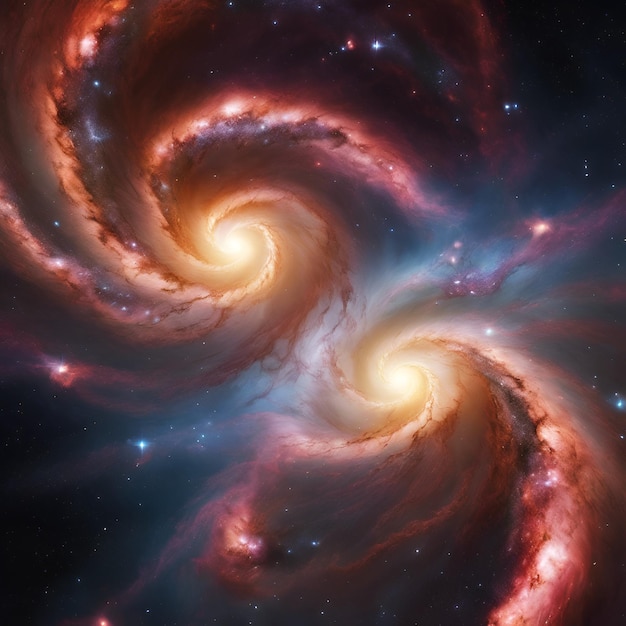The image is an ethereal and powerful digital artwork of outer space, showcasing two galaxies spiraling side-by-side in a captivating symmetry. Each galaxy has a bright yellow nucleus from which spirals of red—almost bloody, creature-like waves of light—emerge, evoking a sense of birth or creation. The red tentacle-like spirals extend vividly against a stunningly dark blue starry background, emphasizing the rapid and dynamic nature of cosmic movements. Amidst the swirls of pink, brown, and purplish hues, twinkling stars add an extra layer of depth, making the galaxies pop against the dark expanse of the cosmos.